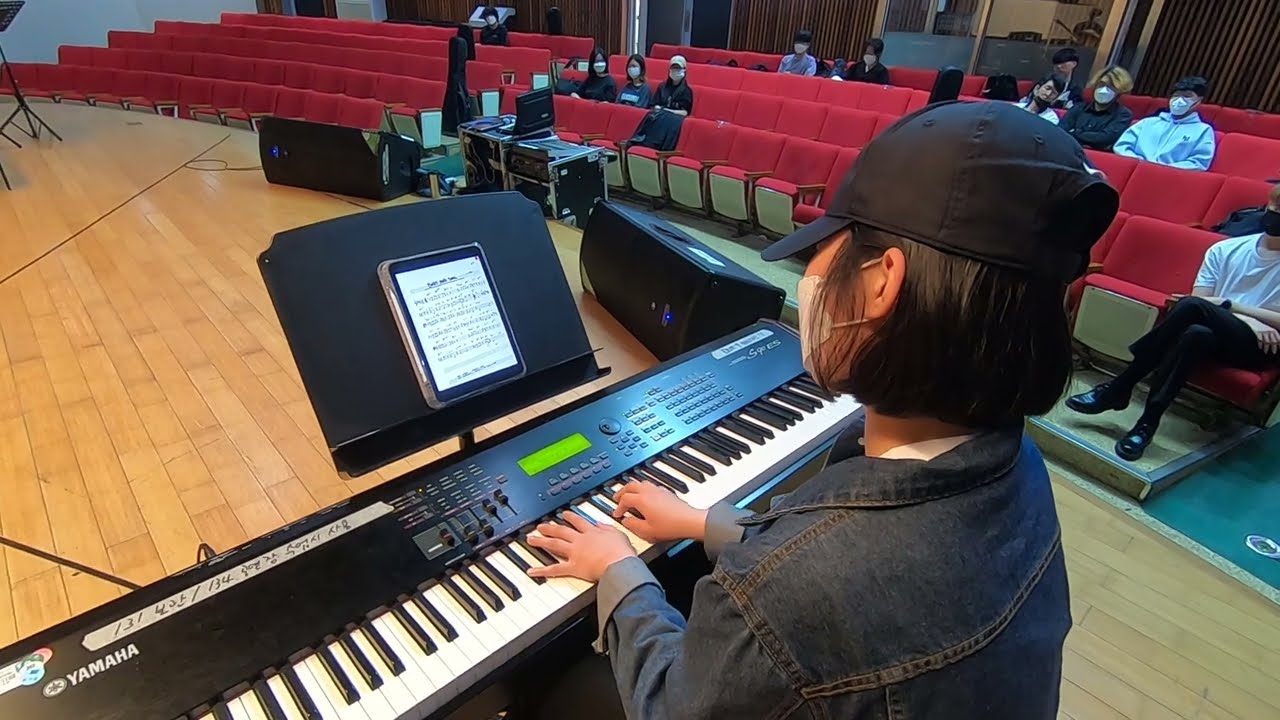The image depicts a young woman seated on a wooden stage, playing a Yamaha keyboard. Positioned over her left shoulder, the keyboard extends diagonally from the lower left towards the upper right at about a two o'clock angle. The woman, identifiable by her shoulder-length black hair, black baseball cap, white COVID face mask, and denim jacket with rolled-up cuffs, has her hands centered on the keyboard. Directly in front of her stands a music stand holding a tablet displaying sheet music. The setting includes two large speakers positioned at the front of the stage. The auditorium, with its red-padded, foldable seats, is sparsely populated; only about 10% of the seats are occupied. In the upper third of the image, small clusters of masked audience members are visible, scattered throughout the four rows of the auditorium. A few individuals are seated in the front and middle rows, while others are dotted along the back row.